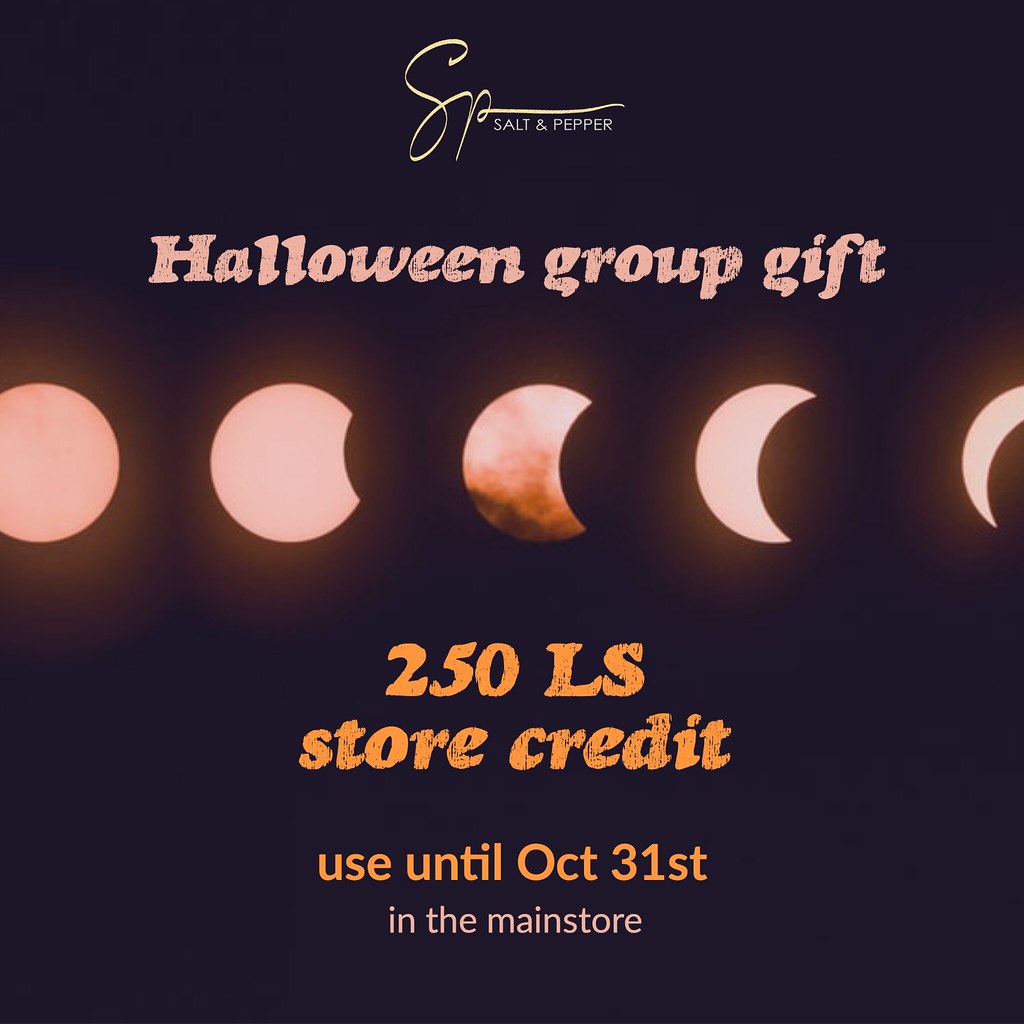The flyer, set against a solid black background, prominently features the SP logo in yellow cursive letters on the top left corner, next to "Salt and Pepper" in small white uppercase letters. Directly below this line, in bold print text, it reads "Halloween Group Gift." The flyer is visually anchored by a sequence of moon phases depicted beneath the text, transitioning from a full moon on the left to a slim crescent on the right. Each lunar phase is slightly cut off by the edges of the image and surrounded by a faint, orangish glow. Below the moon phases, two lines of orange text state "250 LS Store Credit," followed by another line in orange declaring "use until October 31st." The final line, in pink text, indicates the use is valid "in the main store." The text elements are all centrally aligned, enhancing the cohesive, eye-catching design of the flyer.